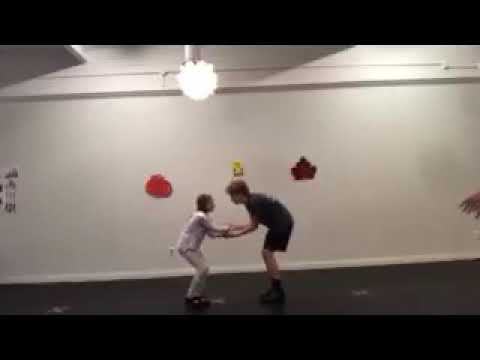In this very blurry and somewhat poor-quality photograph, two figures stand at the center, facing each other with their arms and hands touching as if engaged in a dance or martial arts practice. The setting appears to be a classroom, possibly for dance or karate, with dark hardwood flooring marked with white X’s. The person on the right is notably taller and dressed in a dark t-shirt and shorts, while the shorter individual on the left wears a white short-sleeved shirt, light jeans, or white pants, and dark shoes. Both figures are hunched over, bending at the knees, and looking directly at one another. The background is predominantly white, adorned with ambiguous objects resembling vegetables and other shapes, and a singular, globe-like ceiling light illuminates the scene.